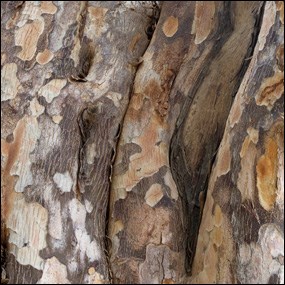This close-up photograph, framed by a thin black border, captures the intricate details of a tree trunk's bark with striking clarity. The textured surface of the bark reveals a patchwork of earthy hues, including browns, reds, and whites, creating a mottled appearance reminiscent of snake skin in certain areas. The bark appears to be in a state of decay, with pieces peeling away to expose the underlying wood in portions. The image is divided into three distinct sections by subtle creases and shadowed gaps. The leftmost section showcases a brownish-gray surface with white and dark brown splotches. The middle fold features a darker gray background with lighter brown splotches and hints of reddish-brown near the top. The right section mirrors the dark gray background of the first, accented by light brown, reddish-brown, and white splotches. Throughout, the bark’s characteristic lines and folds are apparent, with various shapes - circles, ovals, and abstract forms - dotting the surface, adding to the rich, multi-colored texture of the tree trunk.